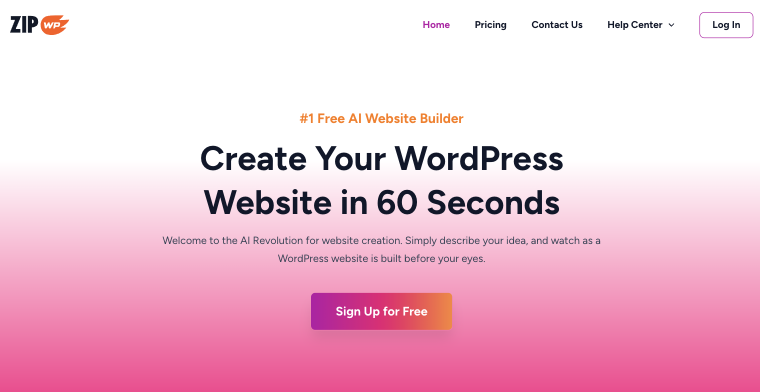The image depicts a web page designed with a gradient color scheme transitioning from pastel pink at the center to progressively darker shades of pink towards the bottom. In the upper left corner, the word "ZIP" is prominently displayed in black. Adjacent to it, there's an orange fire icon with the letters "WP" inside it. On the upper right side of the image, a navigation menu is present, featuring links labeled "Home," "Pricing," "Contact Us," "Help Center," and "Login," all in various shades of pink, with the "Login" link accentuated by a pink outline. Dominating the center of the image, bold black text states, "Create your WordPress website in 60 seconds."